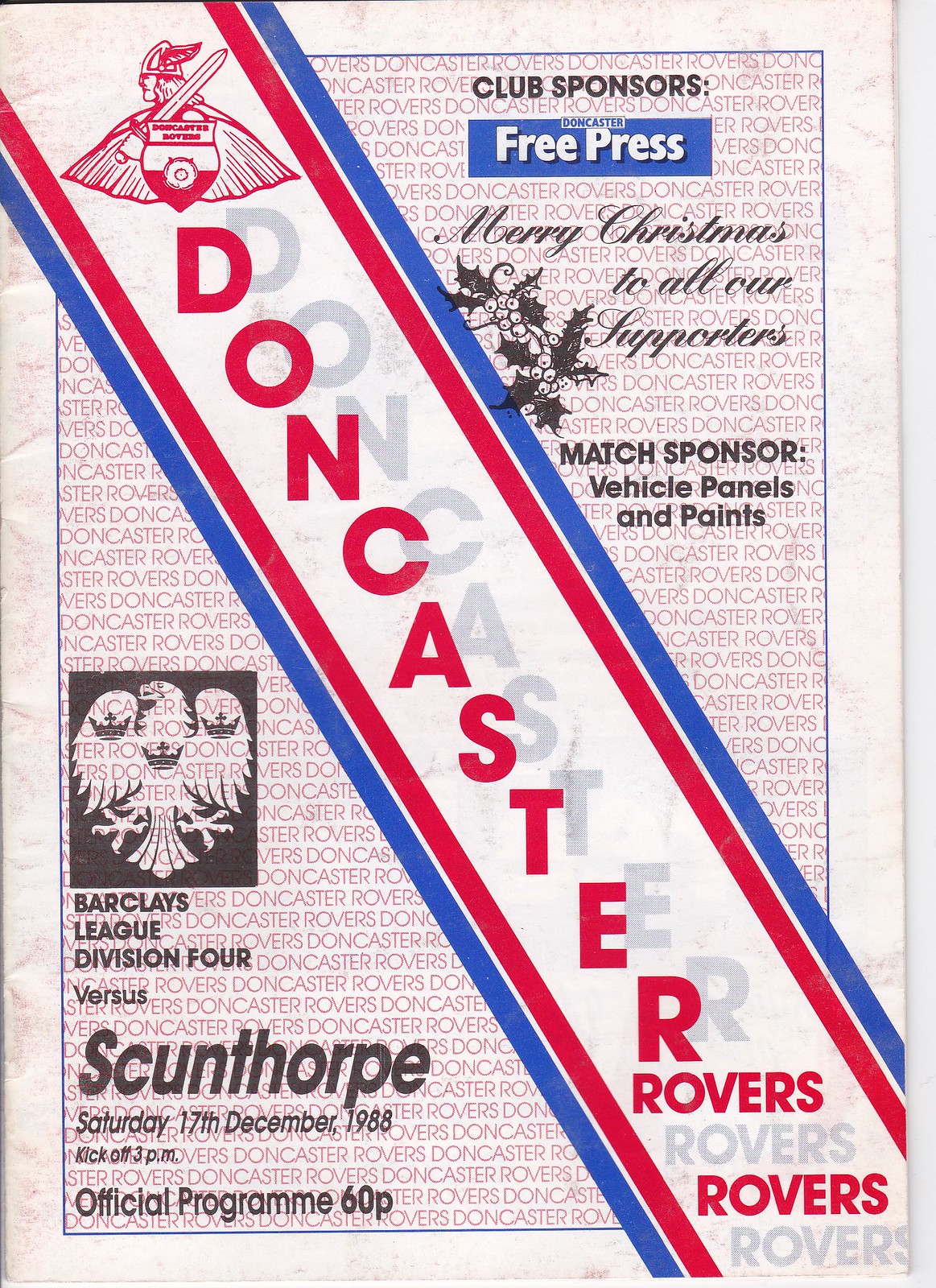The front of the leaflet for Doncaster Rovers soccer team features a background that mimics a weathered white paper with gray stone-like textures, marred by bends and creases, adding to its vintage feel. Diagonally from the top left to the bottom right runs a bold stripe accented with red and blue edges. In the center of this stripe, "Doncaster" is written vertically in red, followed by "Rovers" horizontally in blue. Each letter of "Doncaster Rovers" casts a subtle gray shadow, enhancing its prominence.

Centrally, the background is adorned with a repetitive pattern of "Doncaster Rovers" printed faintly in light red, creating a textured backdrop for the leaflet. At the top, the emblem of Doncaster Rovers stands out—a Viking head facing left with a sword over the shoulder pointing to the upper right, set on a badge with a red base and white middle, all outlined in red ink.

The top right features several notices: "Club Sponsors," "Free Press," "Merry Christmas to All," "Our Suppliers," and "Match Sponsor Vehicle Panels and Paints." On the lower left corner, details of the match are presented, stating "Barclay League Division 4 vs. Grumpthrope, Saturday, 17th December 1988, Official Program Map." Here, the leaflet’s highlights converge, blending the historic and sporty essence of Doncaster Rovers.